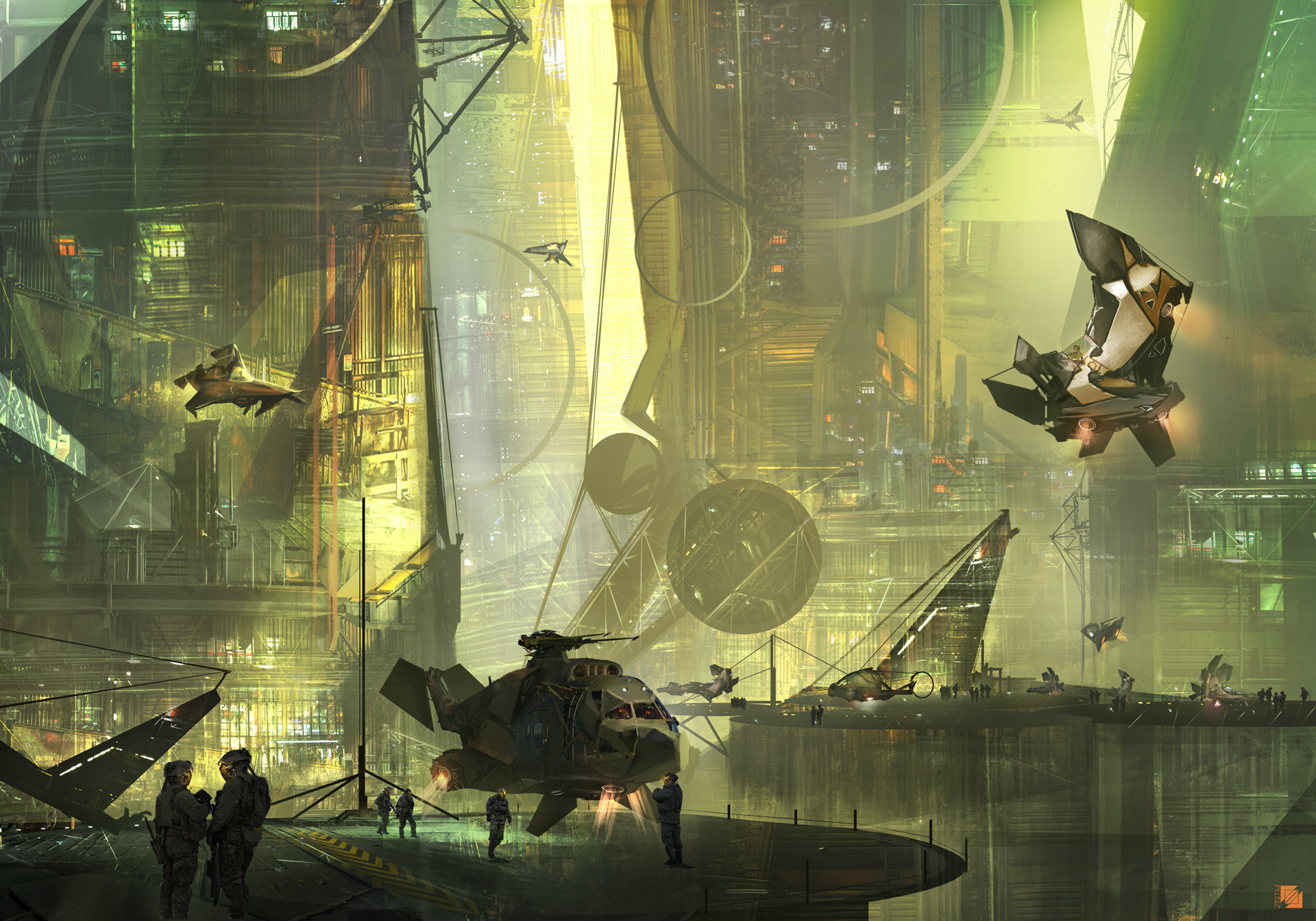In a vividly detailed, computer-generated sci-fi scene reminiscent of futuristic movies or video games, towering, metal-clad skyscrapers dominate the landscape, their armored walls gleaming with a black, shiny hue. This bustling cityscape, bathed in a yellow-green filter, is alive with various futuristic aircraft that resemble modern military vehicles but are distinctly advanced. Among these, a circular-bladed helicopter lacking traditional rotor blades hovers near the front, surrounded by several crew members on a bustling platform. To its back right, another passenger or transport vehicle moves through the air, using thrusters instead of noticeable blades. In the distance, atop another platform, a similar circular-bladed helicopter rests, contributing to the dynamic aerial activity. The left side of the scene reveals a stealth bomber-like aircraft in stealthy black, while the right features a dish-like structure and what seems to be a triangular sail being raised by a rope. The setting's ambiance, enhanced by sporadic beams of light from above, merges elements of steampunk and military aesthetics, creating a captivating and busy metropolis reminiscent of the futuristic world seen in Westworld, but with a unique, almost fantasy-driven twist.